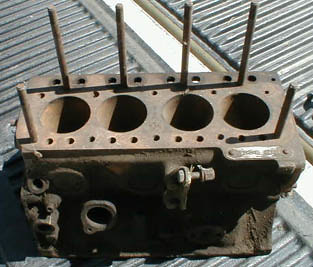The photograph displays a heavily rusted and aged engine block, originally silver in color, evident from the patches of silver metal still visible beneath the rust. The engine block, a large rectangular piece of solid metal, has all its movable parts removed, leaving behind its main cast structure. Prominently on the top surface, there are four circular holes where the pistons would typically be positioned. Additionally, four rods protrude from the top and two from the bottom, which would normally support the attachment of the top of the engine. This engine block is centered in the image and rests on a ridged plastic surface likely belonging to the bed or door of an open pickup truck. The plastic surface displays black and white hues, with a distinct strip of white running between two sections. The scene appears to be outdoors, bathed in bright daylight, emphasizing the contrast between the rusty engine and the somewhat protective truck bed covering.